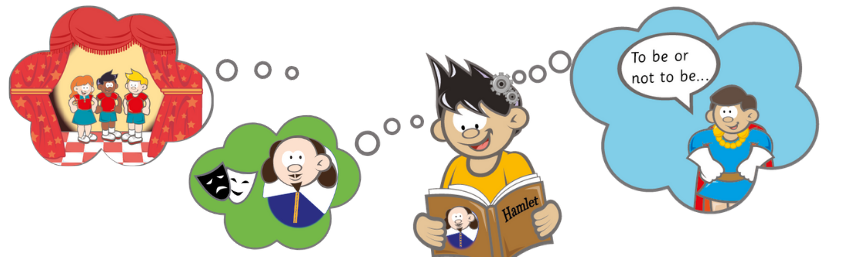The image is a colorful, cartoon-style drawing of a white boy with black spiky hair, wearing a yellow shirt, centered towards the right side of the page. He is engrossed in reading a book titled "Hamlet," which has an illustration of Hamlet on the back cover. Surrounding the boy's head are three thought bubbles, each depicting different aspects of the play he is reading.

On the left, the first thought bubble showcases a stage set with red curtains, featuring three characters performing; they are all dressed in blue skirts or shorts and red shirts. This scene appears to visualize a theatrical performance, potentially an interpretation of a scene from "Hamlet."

The middle thought bubble, slightly to the right of the first, contains images synonymous with theater: a pair of black and white masks representing comedy and tragedy. Additionally, it reiterates the picture of Hamlet from the book's back cover, further anchoring the boy's thoughts on the play's themes and characters.

The rightmost thought bubble shows a character dressed in typical Hamlet attire, with the character pondering the iconic line "To be or not to be," presented in a speech bubble. The background of this thought bubble is a striking blue, contrasting with the greenish hue of the others, highlighting the significance of this famous soliloquy.

Together, these elements illustrate the boy's deep immersion in "Hamlet," as well as his imaginative engagement with the play's dramatic elements.